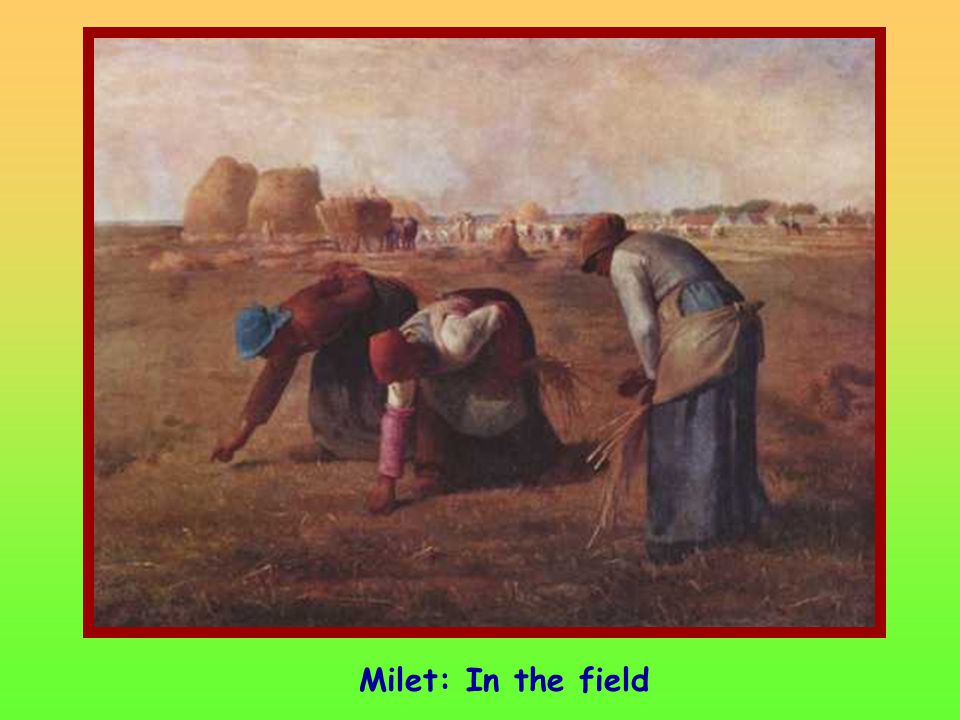A detailed drawing depicts three women laboring in a field, framed by a distinctive red border. Surrounding this red frame, the upper boundary is highlighted in yellow while the lower part is neon green. The women are centrally positioned, each absorbed in picking or examining the ground. The woman on the far left, attired in a blue hat, red long-sleeved top, and a gray long skirt, is bending down with her right hand reaching for weeds. Beside her, another woman dons a red hat and a long skirt with a distinct pink lower-right sleeve, mirroring the posture of the first. The third woman, located to the right, is slightly hunched over, seemingly grasping wheat, and dressed in a brown hat and denim long skirt. Their plain, heavy garments hint at a bygone era. The background features barns on the far left and houses on the far right, with large bales of hay and possibly smoke or low clouds dotting the skyline. The ground beneath them is a uniform brown, emphasizing the fieldwork. At the lower center of the green border, the inscription reads "Millet: Colon in the Field."